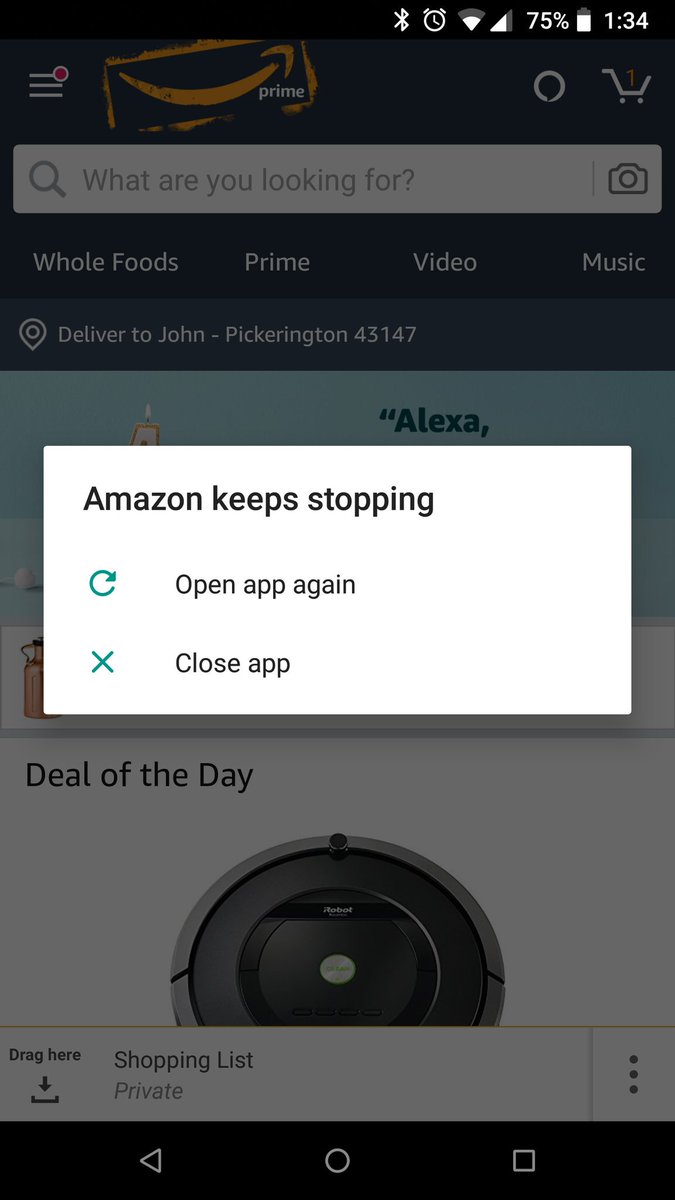This image is a screenshot taken from a mobile device. The foreground prominently displays an error message pop-up from the Amazon app, which reads, "Amazon keeps stopping," with options to "Open app again" or "Close app." In the background, the Amazon app interface is visible, showcasing the search bar along with various categories such as Whole Foods, Prime Video, and Music. The header indicates the delivery address as "Deliver to John, 43147." Additionally, there is a partially visible circular item being browsed or purchased, characterized by a silver outer rim and a black inner section.